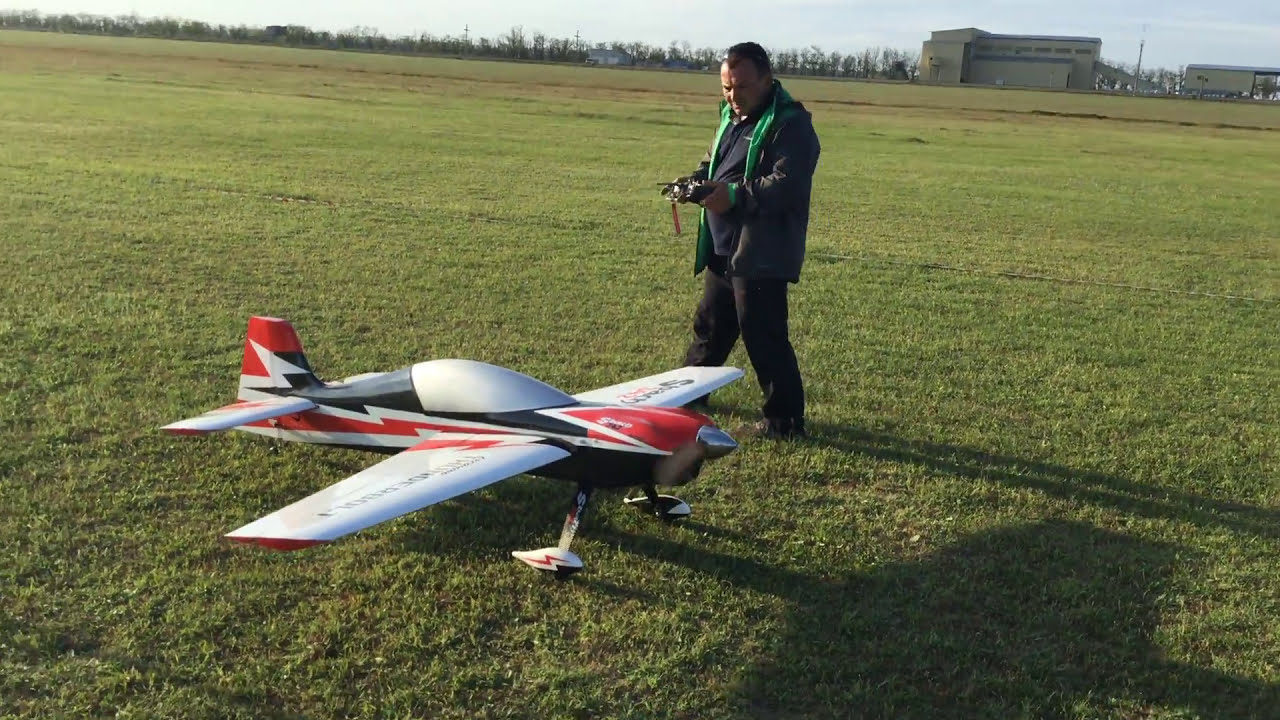In this detailed photographic image, a middle-aged white man is depicted standing alone in a vast, green, grassy outdoor field under a sunny, slightly hazy sky. He is operating a very large remote-control airplane with a wingspan of approximately four feet and a length of about five feet. The man's attire includes a dark jacket with light blue lapels, a blue shirt, and dark pants, and he is seen holding a black remote control. His coat is characterized by shades of green and blue. The striking plane features a silver body adorned with white zigzag lightning bolts and red accents, and the fuselage includes blue sections. Shadows of both the man and the plane are cast on the grassy field. Nearby, a one-story white building that resembles a barn is visible in the background along with a line of trees or bushes, and a couple of other buildings with possibly blue rooftops and either gray or tan siding. The wings of the plane have some text on them, though it is unreadable due to the angle. The entire scene suggests the man is preparing to launch the plane in this tranquil, expansive setting.